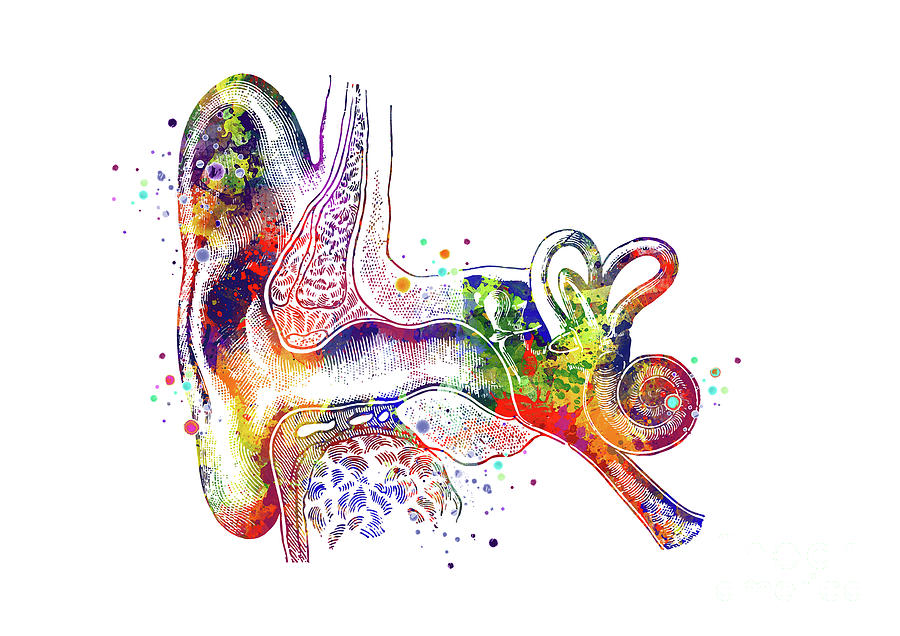The image is a vibrant and abstract rendering of a human ear, utilizing a full spectrum of colors including yellow, green, orange, purple, red, blue, and hints of pink. The piece features various textures and patterns, such as dots and feather-like strokes, adding to its intricate design. The ear, which appears as a zoomed-in and animated object, transitions into different shapes, making it look almost like an animal with visible parts like a backside, paw, and a head with a curled trunk and a heart-shaped form on top. A white streak turns into a rainbow-colored pretzel-like object with red and purple streaks, and a snail-like shell at the bottom. This abstract, multi-colored artwork gives the illusion of movement and transformation, set against a plain white background.